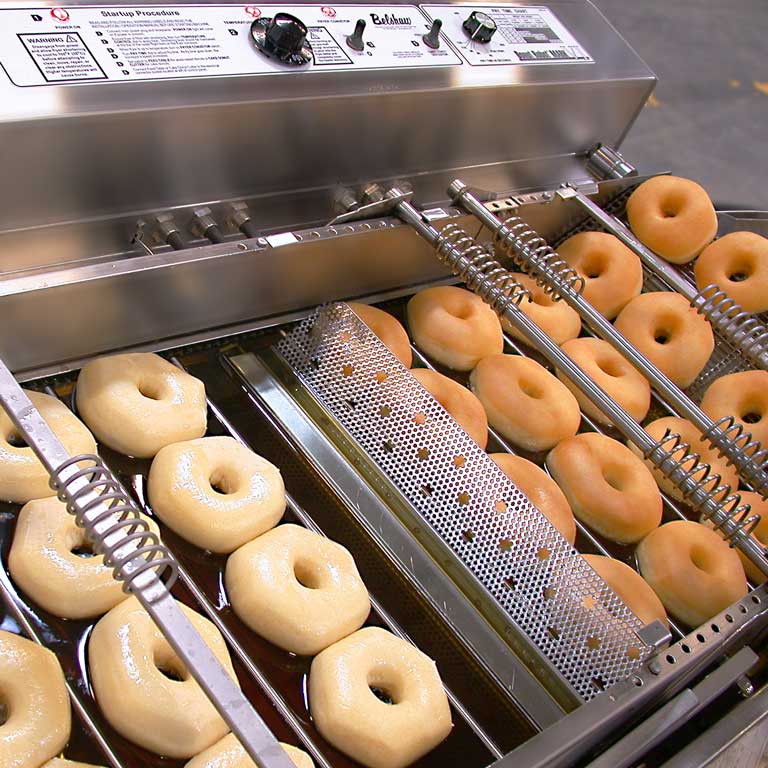The photograph captures the assembly line process of donuts being fried and coated in a sticky substance within a steel contraption. On the left side of the frame, slightly hexagonal raw doughnuts are arranged in rows of four, preparing for their journey. These donuts descend in neat rows beneath the surface of hot oil situated in the midsection of the machine. As they progress through the conveyor system, they emerge on the right side, now perfectly plump, golden-brown, and more rounded. A metal bar structure holds the rows securely in place as they are pushed along.

Above the conveyor belt, a silver metal control panel features an array of dials, switches, printed instructions, and a visible "Startup Procedure" sign. A sticky, brownish substance, possibly honey, coats the donuts as they are lifted from the oil. The entire process is meticulously managed by the machine, which includes grates with star decals positioned atop the donuts. Each row of four donuts sequentially advances through the intricate frying and coating process, ensuring uniformity and quality in each batch. The detailed setup of the machinery, including silver contraptions and safety warnings, highlights the precision involved in producing these delicious treats.